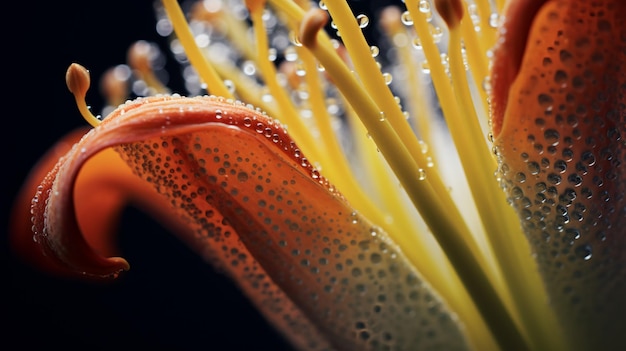This image is a highly detailed macro photograph capturing the essence of a vividly colored flower in stunning focus. At the center of the frame is the main subject – a red flower that almost fills the entire image. The petals of the flower flare out dramatically and exhibit hues ranging from vibrant red to orange, with greens near their base. Scattered across the petals and the flower's central stamen are numerous water droplets, which appear transparent and reflect the red tones of the flower.

The stamen, or the small yellow stems emerging from the flower's core, are delicately outlined and adorned with glistening water droplets, adding a sense of freshness and life to the image. The scene is set against a background that fades into black, emphasizing the flower's vivid colors and intricate details. Some petals curl upwards and others extend towards the edges, with shades transitioning gracefully from red at the tips to the occasional appearance of brown dots on the undersides.

The photograph masterfully captures the contrast between the sharp, focused elements of the flower and the blurred, nearly indistinguishable background. This gives the image a striking clarity and depth, showcasing the minute details such as the water droplets and the texture on the petals and stamens. The overall composition and close-up nature suggest this was taken with a macro lens, highlighting the intimate beauty of the flower in a way that elevates its natural elegance.